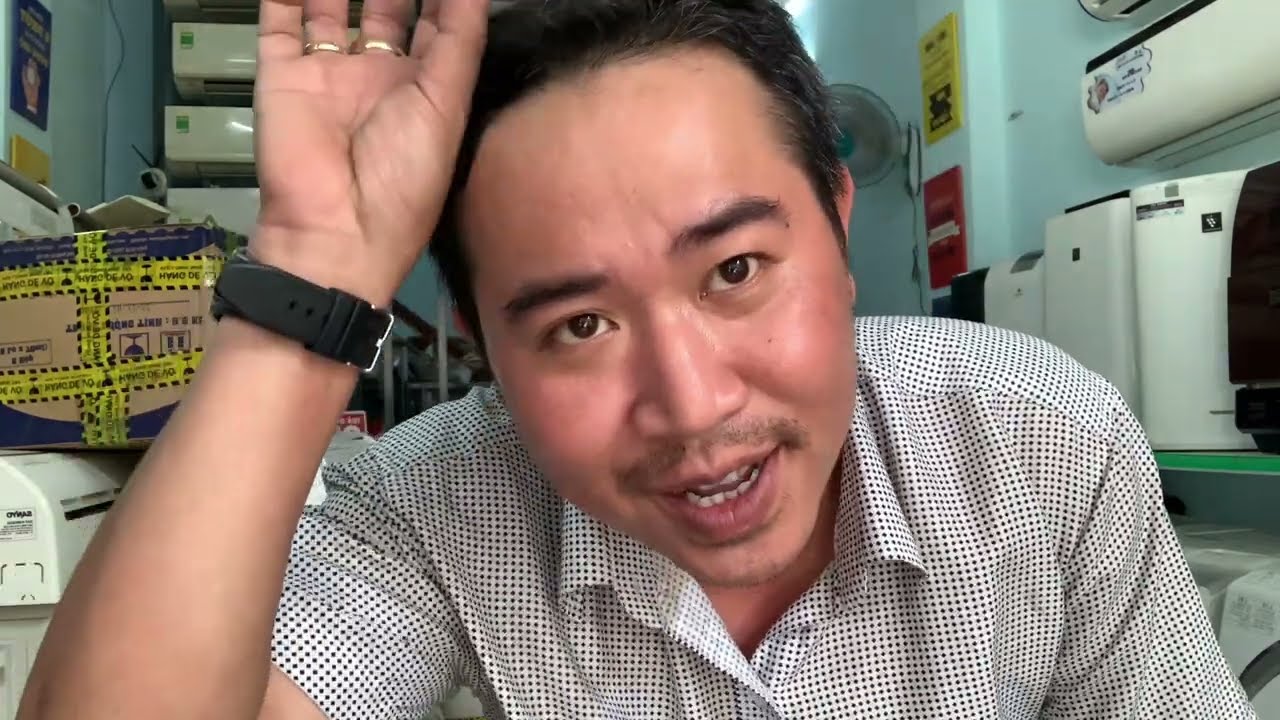The image features an Asian man seated close to the camera, dominating the frame. He has short, dark hair, brown eyes, and is wearing a short-sleeved white button-up shirt adorned with black dots. His right arm is raised with his hand resting atop his head, displaying two gold rings on his middle and ring fingers, and a black watch with its face turned away from the camera. His mouth is slightly open, suggesting he is in the midst of speaking, indicating this could be a frame from a video. The background appears cluttered, resembling an office or storeroom with white walls. Visible behind him are various objects, including a taped-up cardboard box on the left, several white containers, and an air conditioner mounted on the wall. There’s also a small fan positioned higher up, amidst several unidentified electronic appliances that look like small appliances or possibly shredders, adding to the disorganized ambiance of the setting.